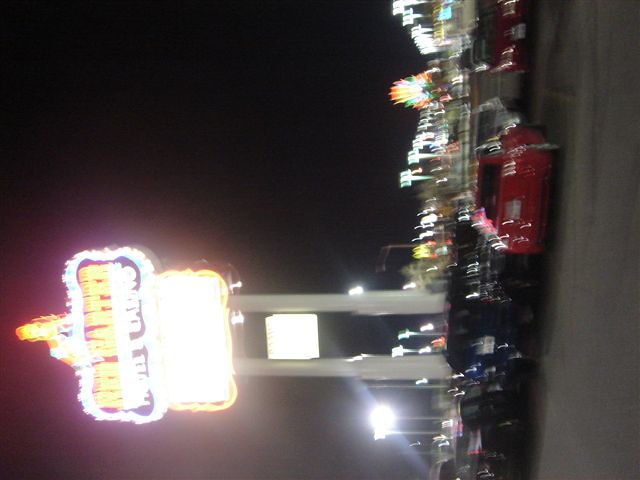The image is a blurry night photo, taken sideways and rotated 90 degrees counterclockwise. The scene appears to be a bustling parking lot, with several red and black cars visible. Dominating the photo is a tall neon sign mounted on two white poles, emitting very bright, vibrant lights. The sign, decorated with pale yellow letters and a rectangular yellow border, possibly advertises a casino. Near the sign stands a tall figure, potentially a cowboy, adding to the casino or western theme. In the background, additional neon lights suggest the presence of other establishments, possibly resembling a setting like Las Vegas, Reno, or Atlantic City. The pitch-black sky and numerous street lamps, along with what seems to be an amusement park ride or Ferris wheel lit in yellow, orange, and green, create a vivid nighttime atmosphere. However, the overall blurriness and motion blur make finer details hard to discern.